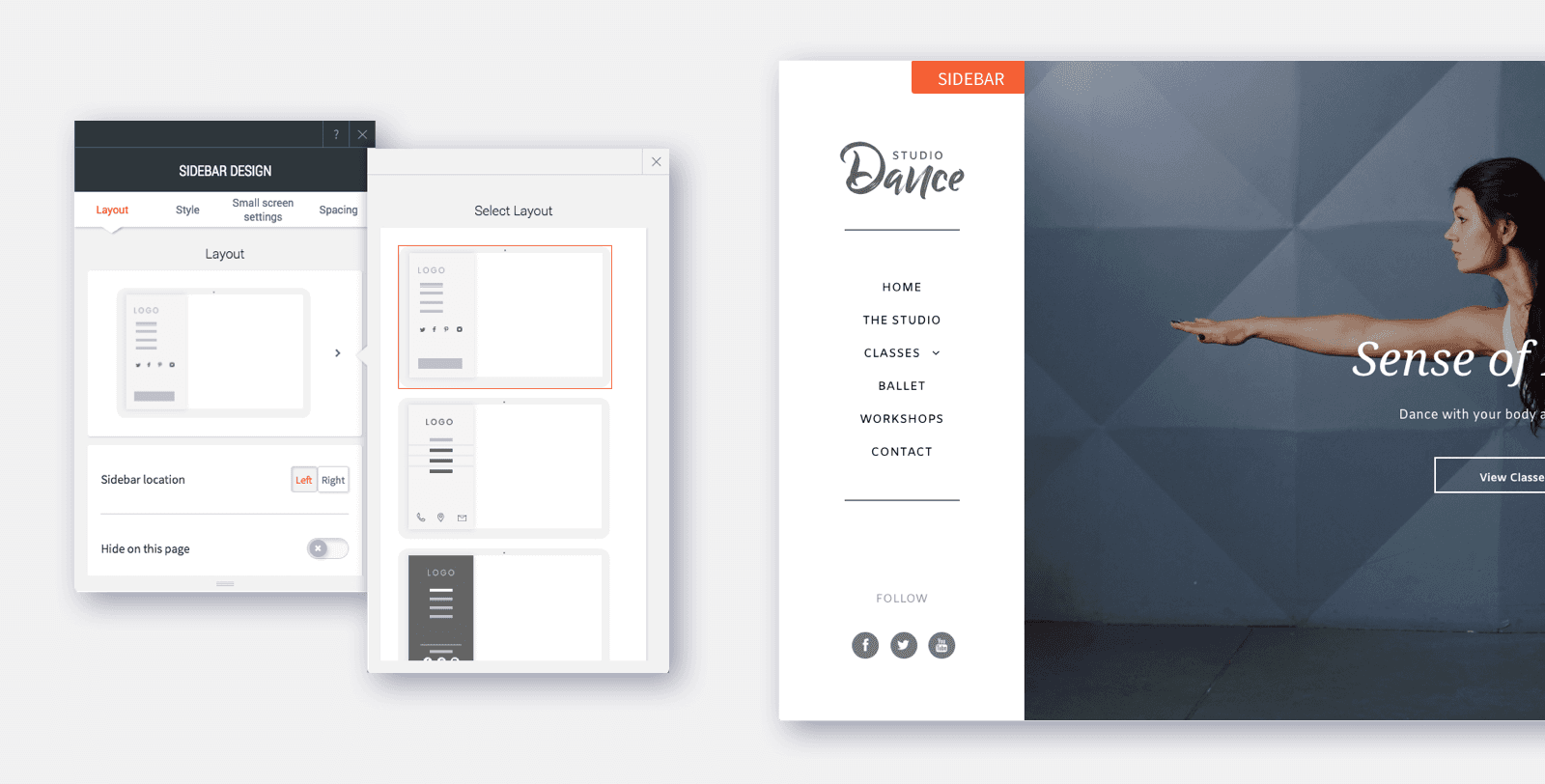The image depicts a website design interface within a design app that allows users to create their own websites. The main image has a light gray to off-white background and features three distinct sections. On the right, there is a standard webpage layout with a sidebar menu that includes options like Home, The Studio, Classes, Ballet, Workshops, Contact, and social media icons for Facebook and Twitter. This section highlights a homepage for "Studio Dance," featuring a professional dancer in profile, extending a muscular arm straight out, with a "View Classes" button and partial text reading "Sense of [something]" and "Dance with your body [something]."

On the left, there are two staggered panels, one of which is a dark gray bar labeled "sidebar design," indicating different layout options. The other overlapped panel with a light gray bar is the active one, titled "select layout." This panel shows various layout options that users can choose from. Both panels suggest tools for customizing the website layout and design elements, with the specific tools indicating that users can personalize their site’s structure and aesthetics. The comprehensive image thus showcases the flexibility and functionality of the web design app.